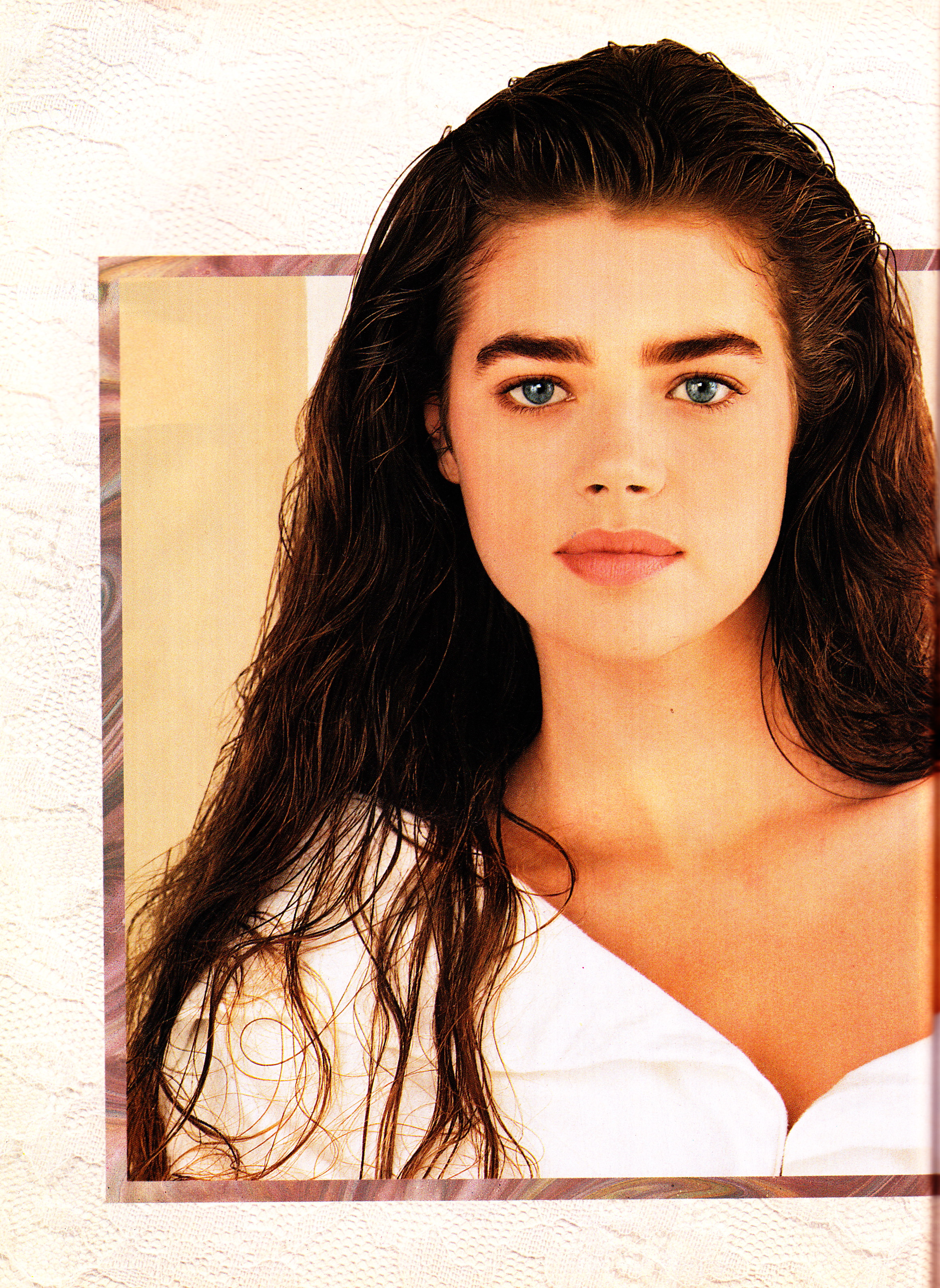The photograph features a young woman who bears a striking resemblance to a young Denise Richards. She has long brown hair, partially draped over her left shoulder while the right side is behind her shoulder. Her eyes are striking, described variably as greenish and bold bright blue, giving her a captivating yet neutral expression that could be seen as deadpan. She has delicate, bubblegum pink lips. The woman is dressed in a white top that is partially unzipped and strategically placed over her shoulders to expose one bare shoulder, creating an uneven neckline that plunges slightly. She appears from her upper shoulders to the top of her head. The image is framed by a border: an outer edge made of white lacy doily cloth material and an inner border of sandstone pinkish gray. Notably, the top of her head extends slightly beyond the frame’s top border. Behind her head is a light beige background, adding to the overall composition of the photograph.